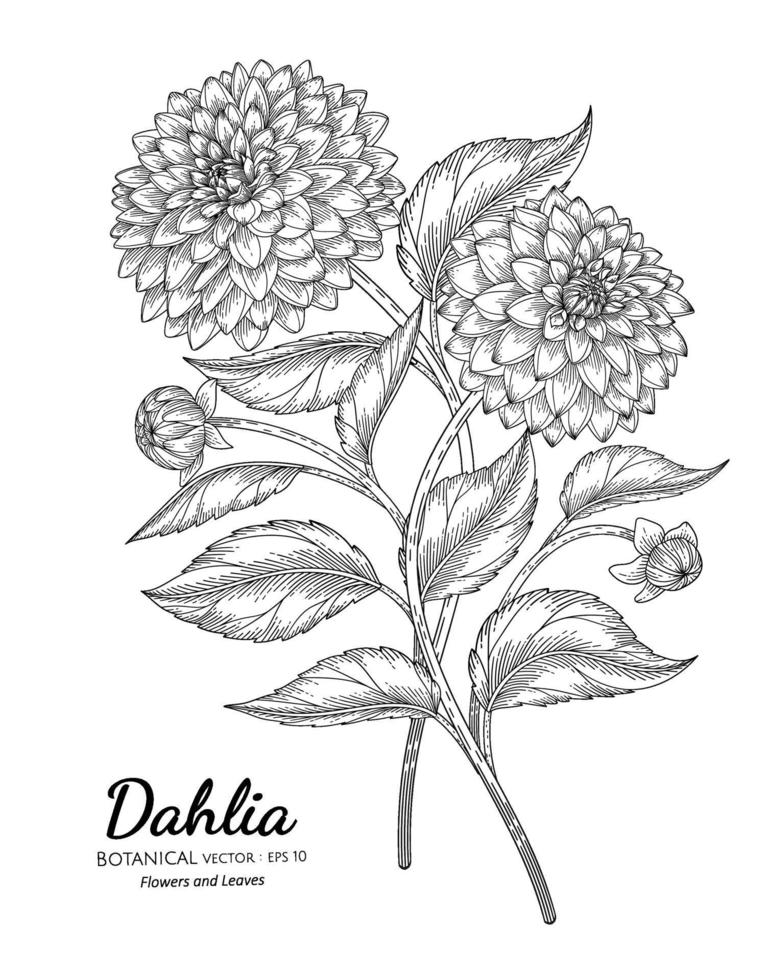The image depicts a detailed black and white vector sketch of a dahlia plant. Central to the composition are two prominent stems, each leading to a large blooming flower positioned at the top of the illustration. Accompanying the blooms are two unopened buds situated lower on the stems. The leaves, characterized by their serrated edges, branch off from the stems and display intricate shading that transitions from the middle of the leaves to their edges. The flowers exhibit similar shading, enhancing their petal structure. Placed against a solid white background, the artwork includes text at the bottom left corner. In bold cursive, the word "Dahlia" is written, followed by "Botanical Vector EPS 10 Flowers and Leaves" in a standard font below. This detailed illustration embodies a botanical style, capturing the essence of the dahlia plant with its blooms, buds, and leaves.